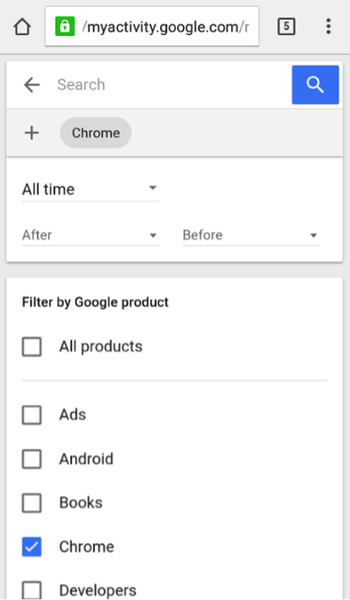The screenshot displays the settings interface of Google My Activity, accessible via the URL myactivity.google.com, prominently shown at the top. Immediately below the URL, there's a search bar for user activity. Underneath the search bar, on the left side, a plus sign is visible, while to the right it reads "Chrome". Following this, the text "All time" is present with an adjacent drop-down menu. Below, within the section labeled "After," another drop-down menu is visible, alongside a similar drop-down for the "Before" section.

The subsequent area is labeled "Filter by Google product," displaying a series of buttons or square icons aligned vertically on the left. Each icon is accompanied by text on the right, listing various Google products, such as All Products, Ads, Android, Books, Chrome, and Developers. Among these, the square for "Chrome" is checked in blue, indicating it is currently selected.